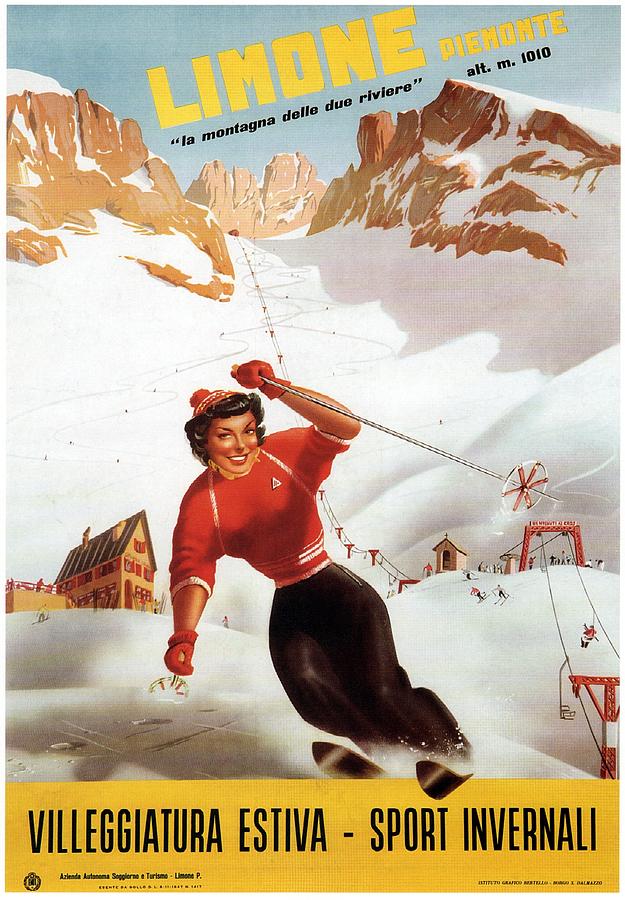The image appears to be an advertisement or promotional poster, possibly from a magazine or for a sports event, and it is likely in Italian. The scene depicts a picturesque ski resort during daytime, featuring snowy mountains with a ski slope running down the middle. At the center, a woman in a red top, red hat, red gloves, and long black pants is skiing downhill while smiling at the camera, angling slightly to the left. In the background, there are several buildings, including a house with an orange facade and a brown roof, and a ski lift with people waiting to ascend. The mountainous backdrop is covered in snow, enhancing the wintery atmosphere. Text in yellow at the top reads "Limon Piemonte," while black text below it says "La Montagna delle Due Riviere." At the bottom, in a yellow banner, it reads "Villa Giartura Estiva Sport Invernale." The vibrant colors of red, black, tan, light brown, brown, and yellow give the image a lively and inviting feel.